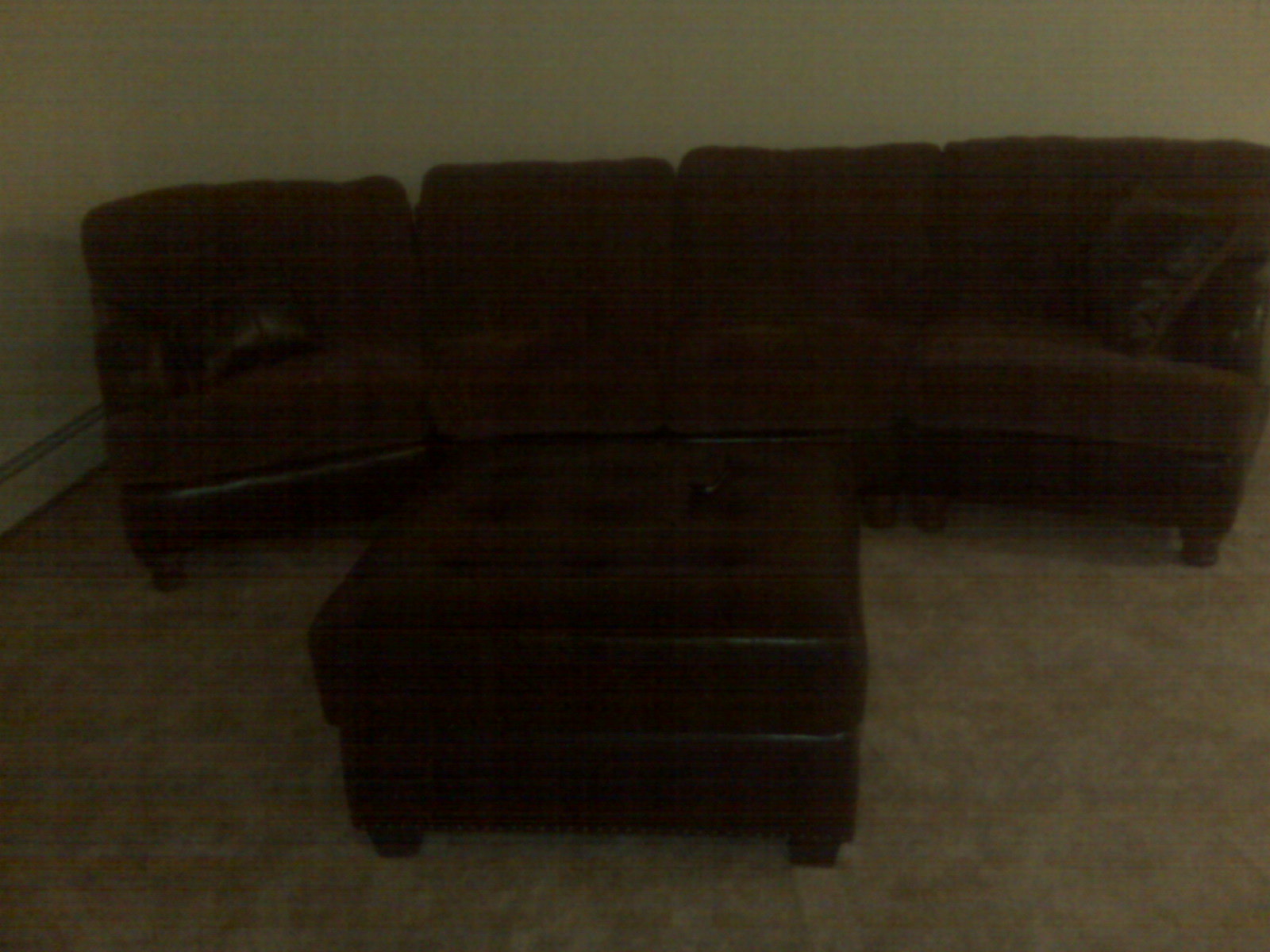The image portrays a dimly lit, grainy photograph of a living room scene featuring a dark brown, leather sectional couch positioned on a dark gray carpet. The sectional is composed of four distinct pieces with rounded legs, suggesting the capacity to comfortably seat four adults. The couch is slightly curved, with the end sections equipped with armrests. In front of the couch stands a large, square ottoman, matching the dark brown leather and material of the sectional. The ottoman, adorned with upholstery buttons on the top and square legs, sits centrally on the floor in front of the couch. The backdrop consists of off-white or cream-colored walls, casting a dim light over the scene which lacks proper illumination. The minimal natural lighting combined with the overall dark tones and graininess of the photo makes the finer details challenging to discern.